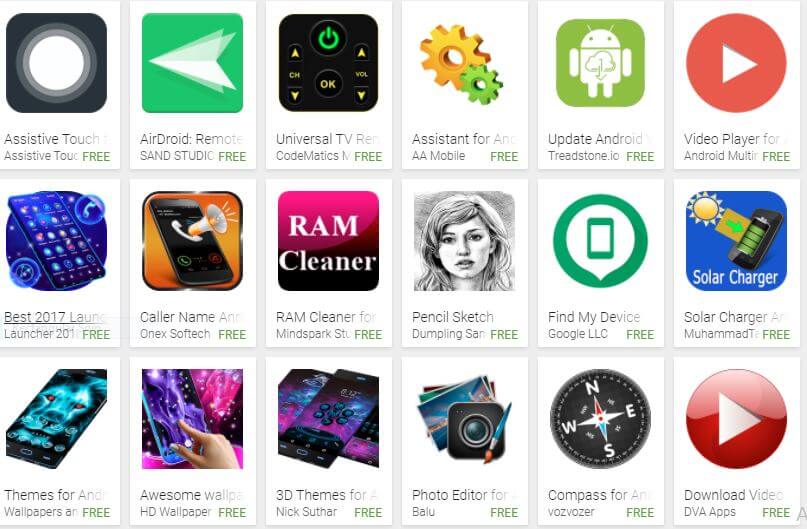This screenshot displays a grid of 18 panel buttons, each representing a different application or tool. Here's a detailed description of the contents, listed from left to right and top to bottom:

1. **AssistiveTouch**: A button labeled "AssistiveTouch."
2. **AssistiveTourFree**: Another button labeled "AssistiveTourFree."
3. **Android Remote**: A green rectangle featuring an arrow, labeled "Android Remote."
4. **SAN Studio**: A black rectangle with a power button icon, labeled "Universal TV Remote" and "CodeMatics."
5. **Assistance for Anne**: Features gears and an Android icon, possibly indicating a utility tool.
6. **Update Android Treadstone**: Displays the Android Robot, labeled "Update Android Treadstone."
7. **Video Player**: A red circle with a white arrow, labeled "Video Player."
8. **Best 2017**: Shows a cell phone icon, labeled "Best 2017."
9. **Caller Name**: A cell phone and megaphone icon, labeled "Caller Name."
10. **RAM Cleaner**: Written in a pink rectangle, labeled "RAM Cleaner."
11. **Pencil Sketch Dumping**: Features a pencil sketch of a woman.
12. **Find My Device**: A green icon, labeled "Find My Device."
13. **Solar Charger**: Displays an icon of the sun and a solar charger, labeled "Solar Charger."
14. **Themes for Anne**: Depicts a blue lion on a cell phone, labeled "Themes for Anne."
15. **Awesome Wallpaper**: Illustrates a space-themed backdrop with colors like purple, pink, turquoise, and black, labeled "Awesome Wallpaper."
16. **3D Themes**: Portrays several cell phones with different themes, labeled "3D Themes."
17. **Photo Editor**: Features an icon of a camera lens and a paintbrush, labeled "Photo Editor."
18. **Compass for Android**: Depicts a compass, labeled "Compass for Android."
19. **Download Videos**: A red oval with a white play button, labeled "Download Videos."

Each icon is visually distinctive, aiding in easy identification of their respective functions, offering a mix of utilities, customization tools, and multimedia applications.